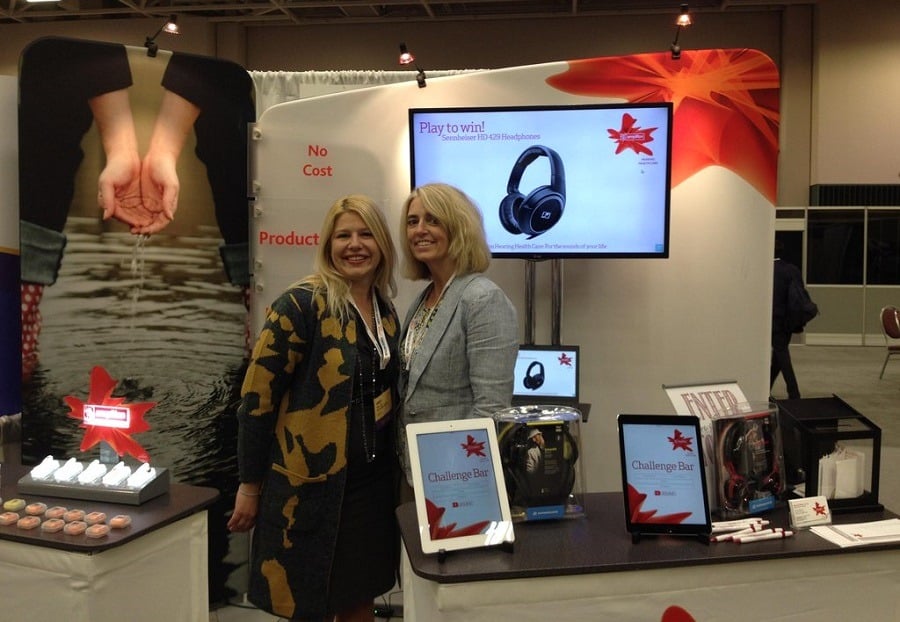This detailed photograph captures a bustling indoor scene, likely taken at a large store or convention booth. Two women with blonde hair are standing side by side, smiling at the camera. The woman on the left, who has slightly longer hair that falls just below her shoulders, is dressed in a black and orange jacket and wears a lanyard with a badge. The woman to the right sports a gray business jacket and has hair that reaches her neck. In front of them, a desk displays two tablets emblazoned with the words "Challenge Bar," one in white and the other in black. Additionally, there is a pile of pens and some business cards on the table.

Behind the women, a wall-mounted monitor and a laptop both prominently display an image of black headphones accompanied by the tagline "PLAY TO WIN" in red. To the left of the monitor, the wall features the words "NO COST" in red and "PRODUCT" directly below. Another noticeable element in the background is a picture of hands pouring water. The atmosphere suggests a promotional or sales environment, with the presence of various electronic devices and promotional materials supporting this notion. The dark exterior visible through the windows contrasts with the bright, engaging setup inside, enhancing the overall impression of a professional and dynamic space aimed at attracting and engaging customers.